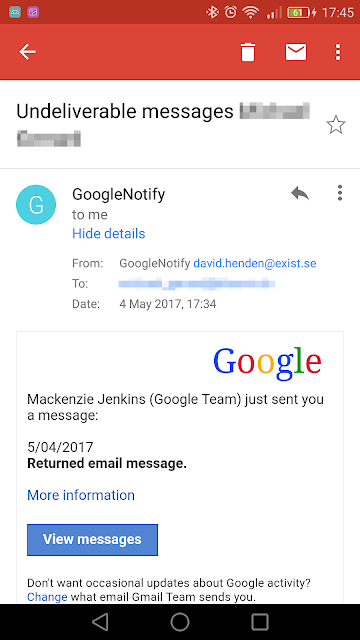The image appears to be a screenshot of a smartphone or tablet display, identifiable by the status icons at the top. The battery is at 61%, the time is 7:45, and there are icons for Wi-Fi, clock, alarm, and Bluetooth connectivity.

The main interface features a predominantly white background with black text, mixed with elements in blue and gray. At the top of the screen, a red bar includes a white back button, a trash can icon, an envelope icon, and a menu with three dots.

Below this red bar, the content resembles an email app. The message section reveals an undeliverable notification from Google. A star icon precedes the sender information, which reads "Google Notify" followed by a partially blurred email address (likely david.henden@exist.se). The timestamp indicates it was sent on May 4, 2017, at 17:34.

The message itself states, "Mackenzie James from the Google team just sent you a message on 05/04/2017 regarding a returned email." A blue highlighted line offers more information, and there's a clickable blue button labeled "View Messages."

Further down, a notification reads, "Don't want occasional updates about Google activity? Change what email the Gmail team sends you."

The interface also includes a turquoise circular icon with a 'G' in it, commonly associated with Google.

At the bottom, standard Android navigation icons are present, including a back arrow, a home symbol, and a recent apps button.